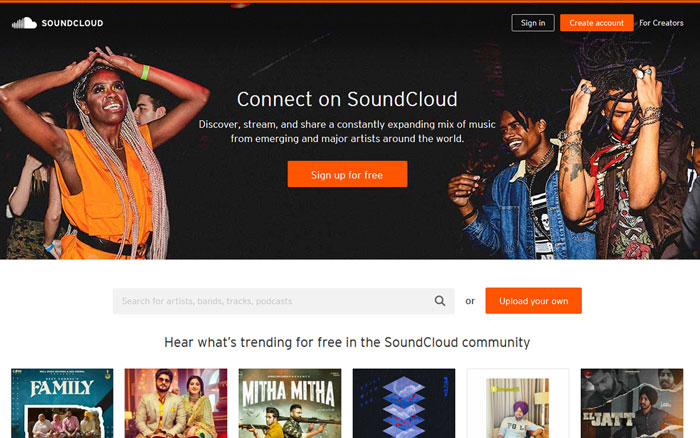The image features a promotional banner for SoundCloud. The top section contains an orange box with the SoundCloud name and icon prominently displayed on the top left. Next to it, there are options for "Sign In" and "Create Account." Additionally, there is a header that says "For Creators."

Beneath this, a text block reads: "Connect on SoundCloud. Discover, stream, and share a constantly expanding mix of music from emerging and major artists around the world." Just below this text, there is an orange button labeled "Sign Up for Free."

The central part of the image shows a group of people who appear to be in a club setting. One individual is wearing a blue jean jacket, another has long dreadlocks, and a third person sports blonde braids that extend past their waist.

Underneath the group image, a search bar is displayed with the placeholder text, "Search for artists, songs, tracks, podcasts or upload your own," followed by an orange search button. Below the search bar, there is another line of text stating, "Here are trending tracks in the SoundCloud community." This section is accompanied by six individual boxes, each containing thumbnails representing different trending tracks.